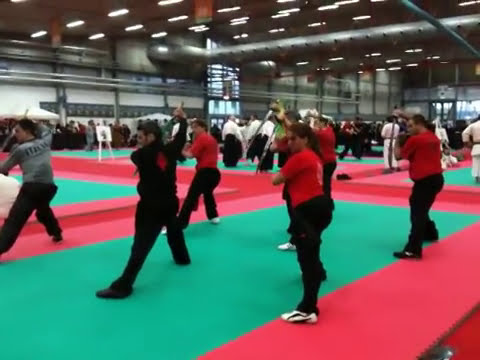In this indoor gymnasium or workout area, a large group of individuals, both male and female and possibly above the age of 30, are engaging in martial arts practice. The scene is set atop a surface with large red mats overlain by smaller green mats, creating a pattern of red rectangles with green rectangles in the middle. At the forefront, approximately eight people are visible, primarily dressed in red shirts and black pants, with exceptions in gray and black attire. They all stand with their legs apart and arms in a unified pose, suggesting they are learning a new move or stance. The space is large and well-lit, with more than 30 visible lights illuminating the area from the gray and silver ceiling above. In the background, another group of individuals in white uniforms is also practicing, contributing to the organized, disciplined atmosphere. Additional details in the far background include a painting or photo atop a wooden stand, integrating an element of decor or inspiration into this vibrant training scene. The image appears somewhat pixelated, likely due to being a screenshot from a video, yet it effectively captures this dynamic and structured environment.